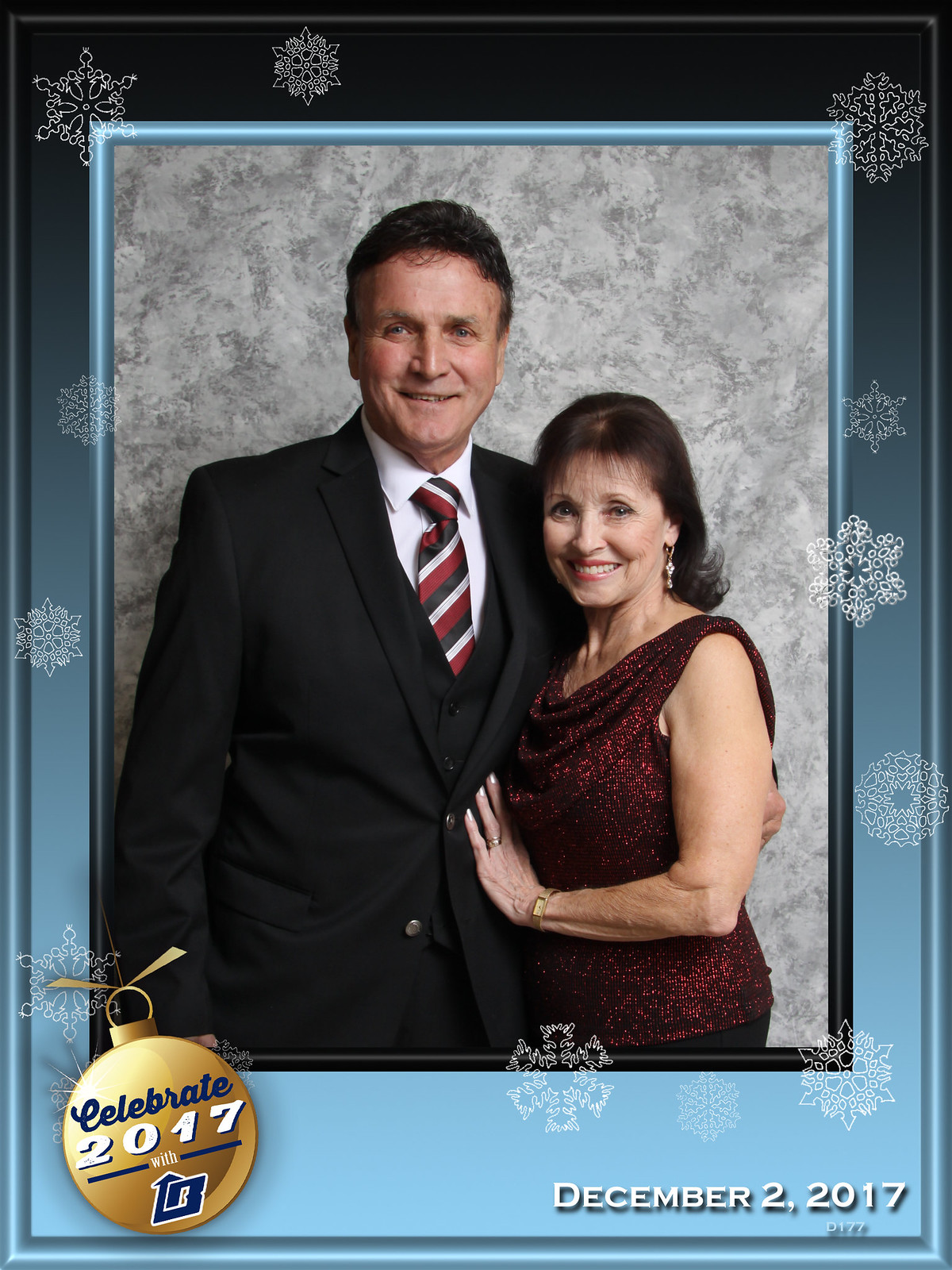This photograph captures an elegant elderly couple posed in front of a gray backdrop. The man, standing to the left, is dressed in a dark three-piece suit, with his vest visible underneath a white collared shirt. He accessorizes with a black, white, and red striped tie. He has a lighter skin complexion and short dark hair. The woman beside him, with her hand resting on his waist, wears a sleeveless, sequined cranberry-colored top with a cowl neckline and dangle earrings; her dark hair reaches her shoulders. They are framed by a border that transitions from black at the top to icy blue at the bottom, adorned with white snowflakes. On the bottom right, the date "December 2nd, 2017" is printed in white. In the bottom left corner, there is a gold Christmas ornament alongside the phrase "Celebrate 2017 with" followed by a logo featuring a bee.